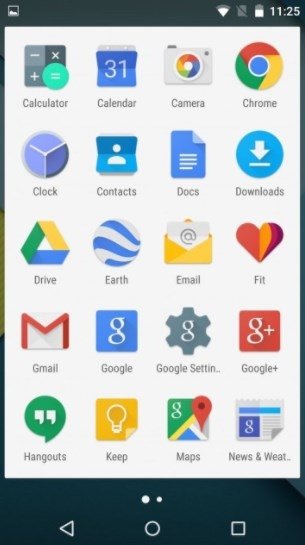This image depicts a smartphone screen in vertical format, showcasing a variety of app icons commonly found on such a device. At the top right corner, the screen displays the time, Wi-Fi signal, and battery status symbols. Below these indicators, a host of app icons are neatly arranged.

Among the icons, there is a calculator symbol, a calendar icon displaying the number 31 with plus and minus buttons, and a camera icon featuring a white camera with a colorful lens. The Chrome icon stands out with its recognizable multi-colored design, and the clock icon shows a typical clock face.

Additionally, the contacts icon displays a white silhouette of a person on a blue square background. There is also an icon for Google Docs labeled "Docs" in blue, along with a downloads icon, followed by Google Drive. Another app indicated by a globe icon with blue lines represents Google Earth.

The email app icon appears as an envelope, accompanied by a fitness app symbolized by a heart. The Gmail icon is another envelope, but distinctly marked. For general Google services, a white "G" is displayed, as well as a Google search icon. The settings are represented by a gear icon, and Google Plus is depicted with a white "G" and a plus sign.

Also visible are icons for Hangouts, Google Keep, Google Maps, and a news and weather app, completing the array of standard smartphone applications on this screen.